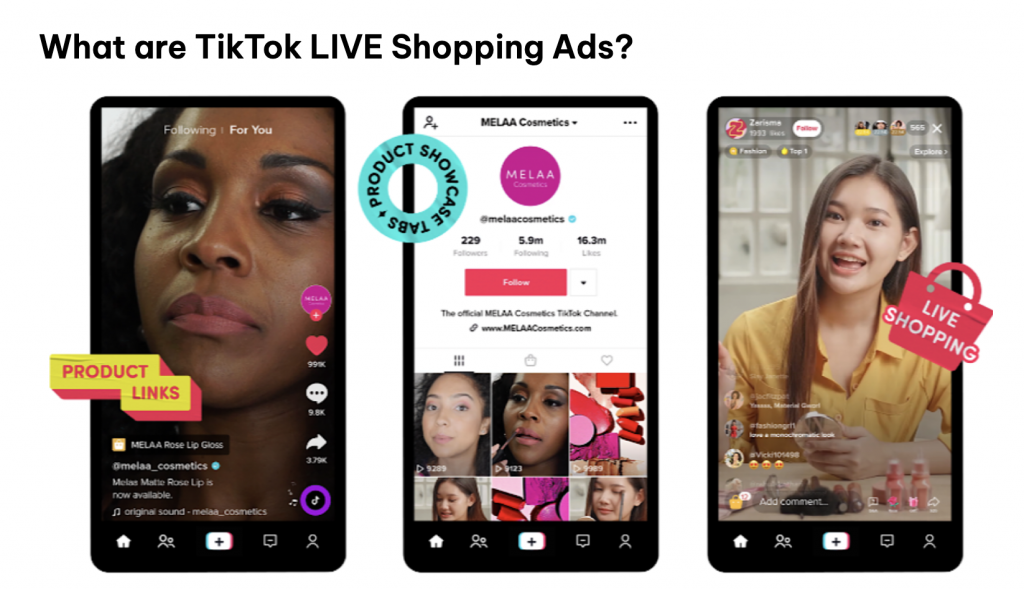A detailed screen capture features three simulated cell phone interfaces illustrating TikTok live shopping ads. At the top, a black header raises the question: "What are TikTok live shopping ads?"

The first phone screen displays a dark-skinned woman donned in mauve lipstick and orangish eyeshadow with thick black lashes. Prominently positioned over her forehead are the categories "Following" and "For You." Below, "Product Links" is highlighted in a mix of green and pink text. The interface also showcases several icons: a purple-pink circle, a red heart, and a white speech bubble icon among others. The description reads "Mila Rose Lip Gloss" from the handle "@MilaCosmetics." Additional features include a blue circle with white text beneath, a TikTok logo circled in purple, and a consistent set of icons at the bottom for navigation (a white house, cartoon people, a plus sign in a box, a speech bubble, and another cartoon person).

The second phone screen has a predominantly white background, featuring a black cartoon head icon next to "Mila Cosmetics." There are three lines and a light pink circle with white text. A teal and black circle states "Product Showcase." It depicts the account's stats: 229 followers, 5.59 million following, and 16.3 million likes with a prominent pink "Follow" button. A pull-down menu describes "The Official Mila Cosmetics TikTok Channel," followed by a chain icon and link. This screen shows a collage of people applying makeup, red and pink cosmetic products, a shopping bag icon, and the same recurring icons.

The final image presents a brown-haired woman in a yellow-gold shirt, seated at a table with various cosmetics in front of her. Interactive elements such as user comments are visibly popping up. A pink bag icon with "Live Shopping" in white text denotes the active shopping experience.

Overall, the screen captures provide a vivid depiction of how TikTok integrates product promotions within its live shopping experience, highlighting interface elements, user interactions, and real-time cosmetic showcases.